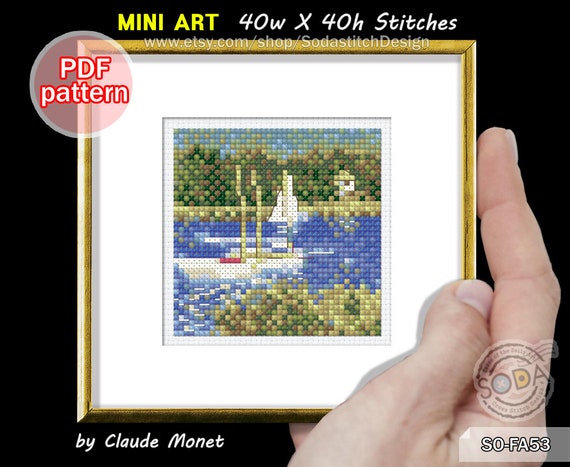The image is an advertisement with a predominantly black background. At the very top, in yellow font, it reads "mini art," followed by "40W x 40H stitches" in white text to the right. Below this text is a watermark that states "www.etsy.com/shop/sodastitchdesign." Just beneath "mini art," positioned at the top left of the image, there is a white circle with a dull reddish-pink center. Inside this circle, outlined in red, are the words "PDF pattern."

The main focus of the ad is a hand holding a very small piece of stitched artwork within a brass-colored frame. The hand appears from the bottom right of the image, with the thumb on the top right corner of the frame and the forefinger on the side. The artwork within the frame shows two boats on a lake, surrounded by trees and a shoreline with bushes or grass. The image appears pixelated, emphasizing its stitched nature. At the bottom right corner of the frame, the text "by Claude Monet" is visible. Additionally, there is a round insignia near the bottom right corner, crossing the forefinger, with the word "SODA" prominently visible.